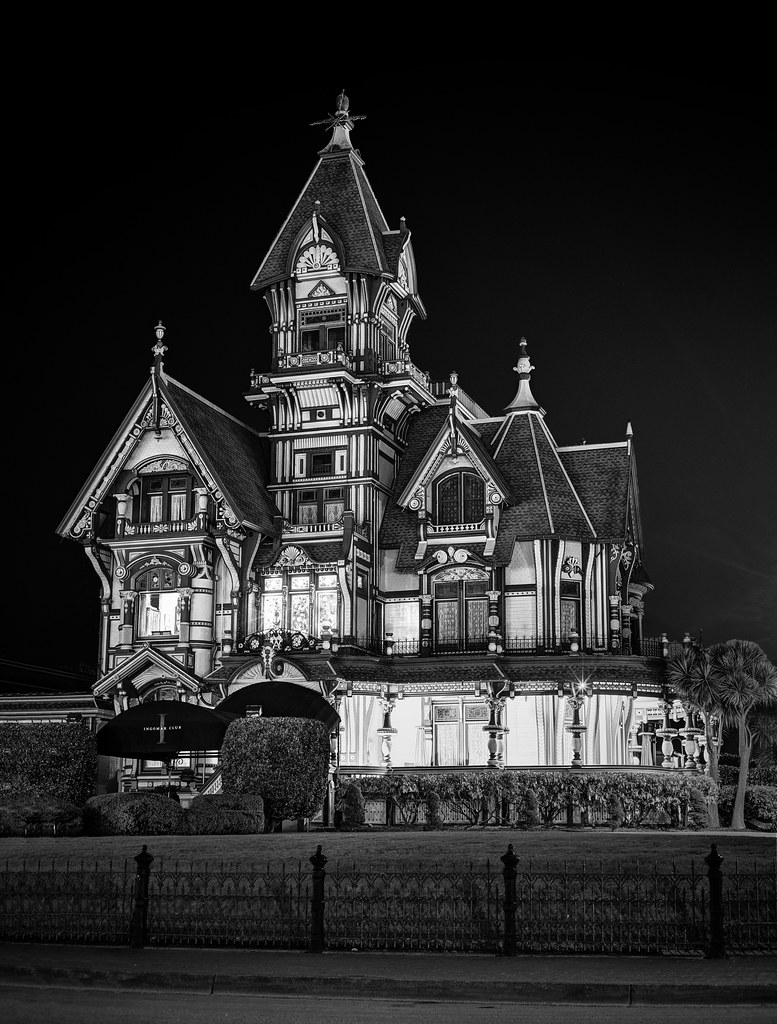This black-and-white illustration is a detailed, portrait-oriented sketch of a large, elaborate house, evocative of Victorian Gothic architecture, resembling the Carson Mansion in Eureka, California. The setting is nocturnal, with a dark night sky providing a backdrop to the intricate structure. The house, rendered meticulously in shades of black, white, and gray, features a central tower that rises at least one floor higher than the rest of the four-story building, adorned with multiple pointed structures and decorative pediments over the windows.

The façade is marked by a round porch that wraps around the front of the building, supported by multiple posts. On the bottom left, a gabled end has a walkout balcony above an arched opening, while to the right, the central entry features a covered porch with double doors underneath an additional walkout balcony. The house is enclosed by a brick wall, with a sidewalk running alongside it, and in the foreground, a row of tailored shrubbery is meticulously noted. The image lacks textual elements, focusing solely on the architectural beauty and historic ambiance of the depicted structure.